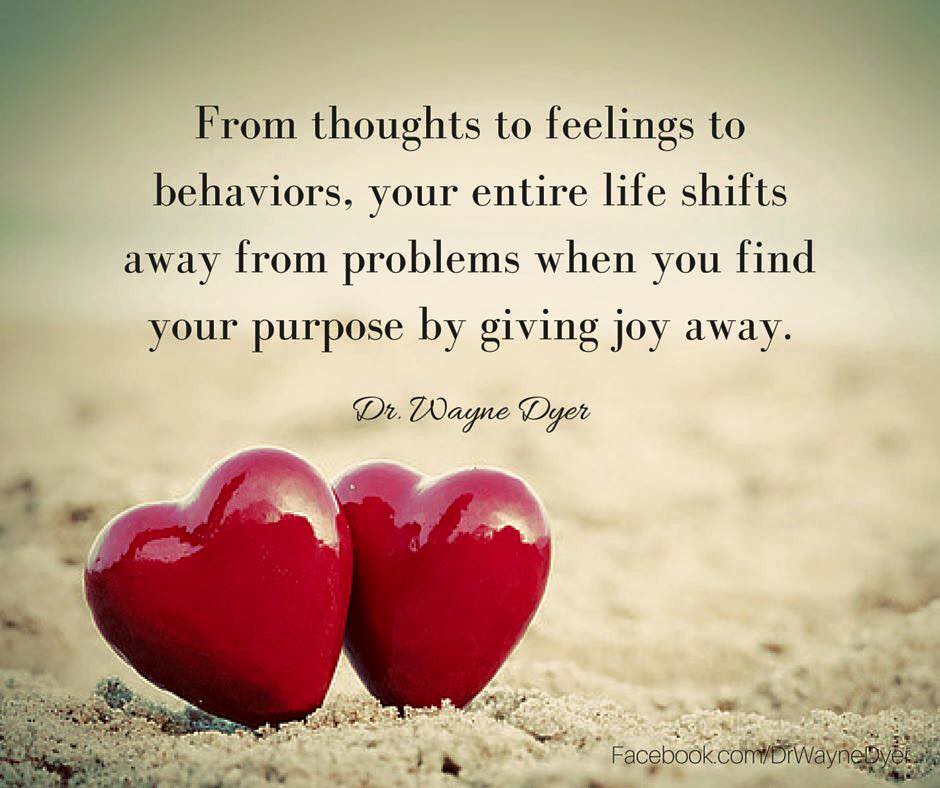This is a computer-generated image featuring an inspirational quote. The scene appears to depict a beach or a desert, with sand dominating the lower two-thirds of the frame. The background is hazy, possibly hinting at an ocean or more sand falling away into the distance. In the bottom left-hand corner, two red, shiny heart-shaped objects, resembling artistic knick-knacks or candies, are nestled together, contributing to a Valentine's Day theme.

Centered above the hearts, an inspirational quote is displayed in a slightly squished Times New Roman font in black. The text reads: "From thoughts to feelings to behaviors, your entire life shifts away from problems when you find your purpose by giving joy away." Beneath this quote, in cursive, the name "Dr. Wayne Dyer" is prominently displayed. At the bottom right corner, the website "Facebook.com/DrWayneDyer" is written in thin text.